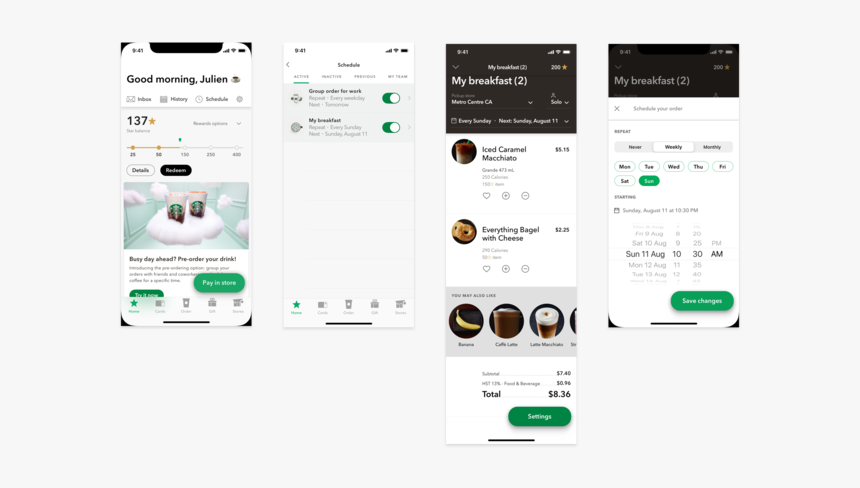In the image, there is a large light blue box containing four smartphone screens displayed in a sequence. 

The first screen features a sophisticated interface with a white rectangular box at the top displaying the text "Good Morning, Julian," accompanied by three small interactive buttons. Within this screen, a value of "137" is highlighted with a yellow star icon next to it. Below, there is a yellow slider button flanked by a white button and a black button. Additionally, an image depicting a cloud with two small phones inside is present. At the bottom, there's a prominent green "Pay" button, a partially visible green button, and a green star within the image's four corners, each containing subtle black sections. The screen is bordered at the bottom by a black line.

The second screen has a minimalistic design with a white background. It displays some text that is partially unreadable, accompanied by two blue boxes and corresponding green toggle buttons. At the base of the screen, there is a green star along with various other icons and a black line.

The third screen starts with a bold black box showcasing the time "9:41" and the text "My Breakfast Too." The screen contains several elements in white print, such as a white rectangular box and images of an iced caramel macchiato, an everything bagel with cheese, and a blue box holding a banana and a coffee cup with whipped topping. It also partially displays another circular item. The total cost highlighted on this screen is $8.36, accompanied by a green settings button at the bottom.

The fourth and final screen presents a clean design with a black section at the top, labeled "My Breakfast Too," including an "X" and an additional box. Below, a white rectangular box shows three buttons aligned at the top, the days of the week with "Sunday" highlighted in green, and the date "Sunday, the 13th August" along with the time "10:30 a.m." A green "Save Changes" button is prominently displayed. Like the other screens, this one also has subtle black corners and a black line at the bottom.